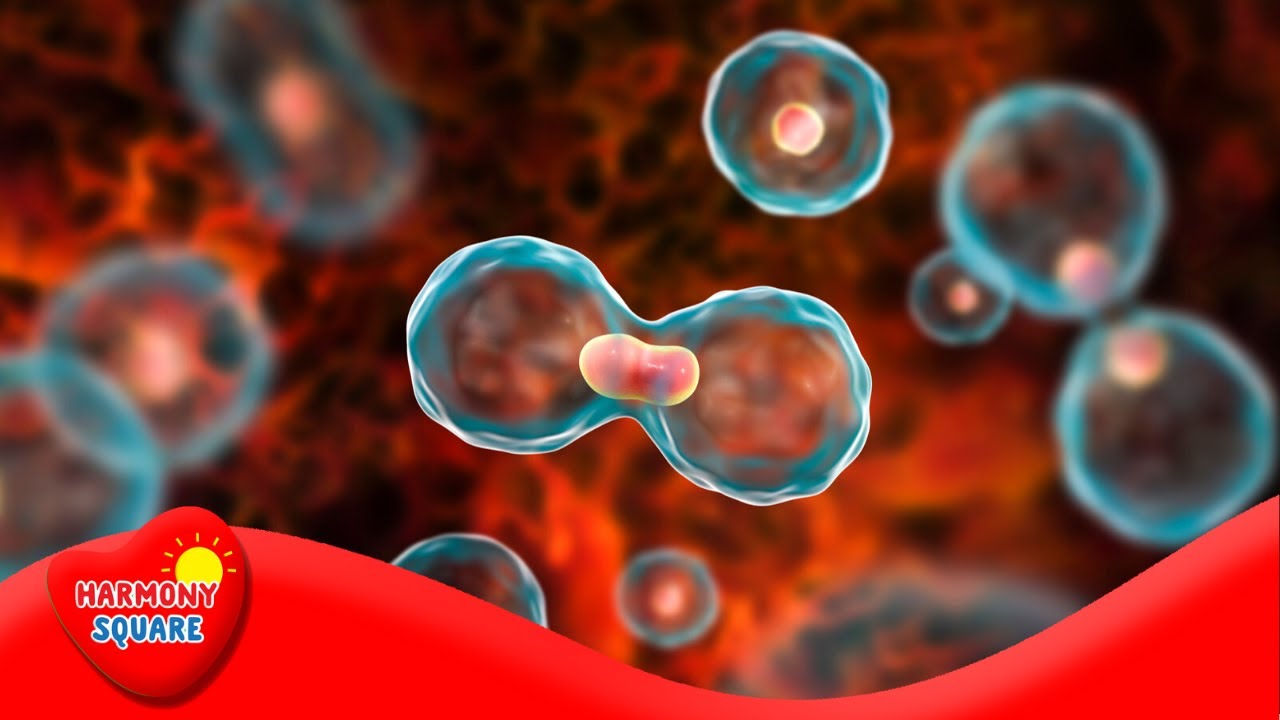The image appears to be either a photograph or a computer-generated illustration, possibly of a microscopic scene or a highly detailed painting, depicting a process that resembles cellular division or mitosis. Dominated by blue bubbles that are shown in various stages of splitting, the image features conjoined circles, often sharing a small pink or red, cylinder-shaped center, likely representing a cell nucleus. Many bubbles are seen fully split, each retaining a part of the nucleus. The background is a vivid red, enhancing the contrast and making the blue structures more prominent.

In the bottom left of the image, there is a distinctive illustration: a yellow sun with radiating lines and a red, wavy heart shape, accompanied by the text "Harmony Square." This logo anchors the piece and provides a branding element to an otherwise biological-themed visual.